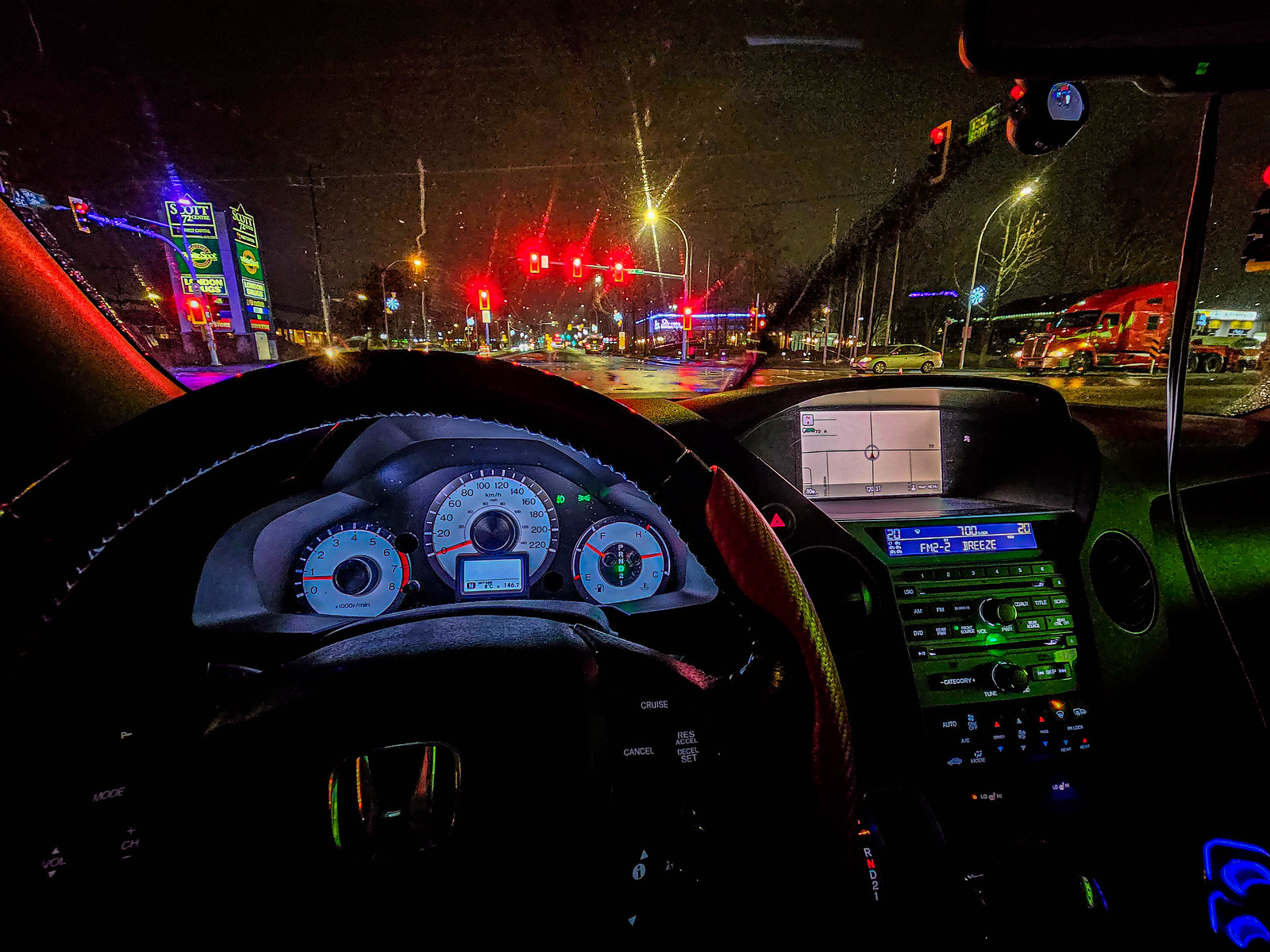This photograph, taken from the driver's seat of a car at night, showcases a detailed interior and exterior view. The bottom half features the car's dashboard, which is partially illuminated. The black steering wheel, accented with patches of brown, occupies the left side. Behind it, three round dials are clearly visible: the speedometer, tachometer, and thermostat. To the right of the steering wheel is the car's radio and air conditioning panel, and above them, in the center of the dashboard, is a built-in GPS navigation system. Through the windshield, red traffic lights are visible in the center, casting a faint glow on the scene. On the left side of the photo, a square sign displaying two sides—a blue background and a green background—is partially visible, giving the impression of a cube. On the far right of the image, the vibrant red and yellow cab of a tractor-trailer truck can be seen. The top portion of the photo is dark, emphasizing the nighttime setting.